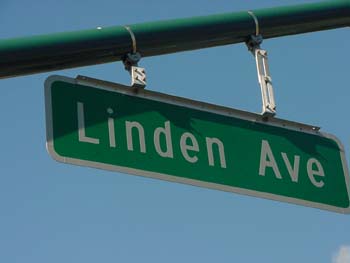The image depicts a square photo featuring a street sign for "Linden Avenue." The rectangular sign itself has a silver border and a green background, with the word "Linden" spelled out in silver letters, followed by the abbreviation "A-V-E" for Avenue. At the top of the sign, two objects are attached and hanging, all connected to a green pole that stretches diagonally from the top left to the top right of the image. The background showcases a light blue sky with a small patch of clouds.